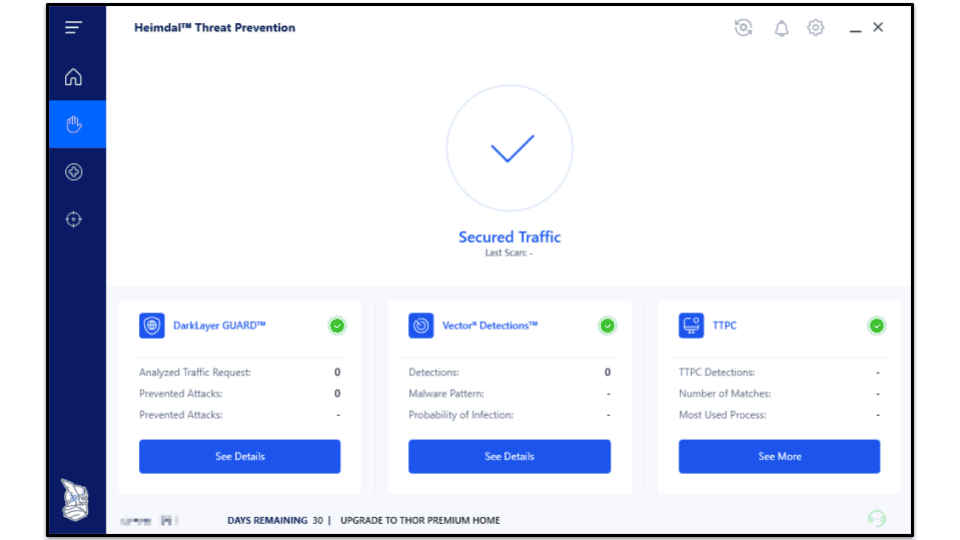This is a horizontally oriented image typical of a webpage layout. The image is framed by a medium black border with a white background in the content area. On the far left of the image, there is a vertical navy blue line that hosts several icons from top to bottom: three horizontal lines (presumably a menu icon), a home icon, a hand icon, a plus button, a compass or search icon with a central dot, and a white emblem at the bottom.

In the upper left corner of the white background, the text "Heimdall Threat Prevention" is prominently displayed. In the upper right corner of the white section, there are additional icons including a refresh or switch button, a bell, a settings gear, a minimize button, a close button, and a light blue circle with a dark blue check mark inside it, which is bordered in white but not filled in. Below this circle, blue text reads "Secured Traffic, Last Scare."

Centered in the image are three white boxes with blue square icons: the first labeled "Dark Layer Guard," the second "Vector Detections," and the third "TTPC." Each of these boxes provides some information about its respective feature, with a blue button beneath each one labeled "See Details."

At the very bottom of the image is a gray strip containing the text "Days Remaining: 30 Upgrade to Thor Premium Home."